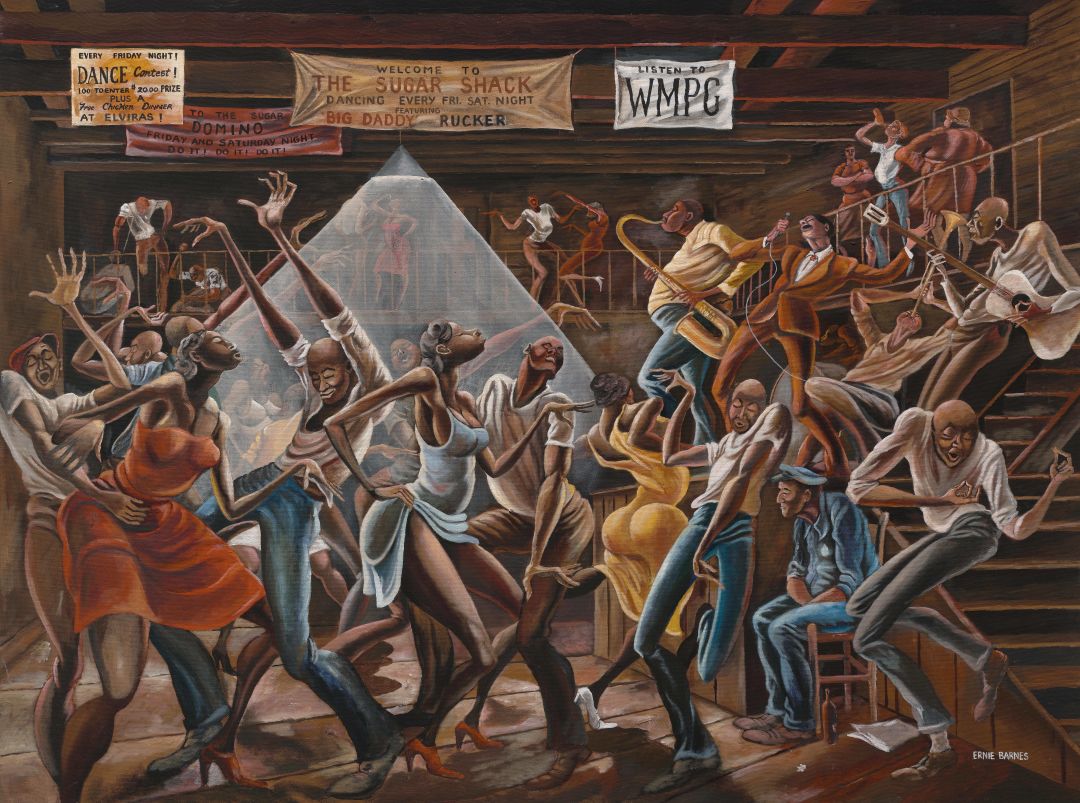The image is a colorful painting depicting the inside of a bustling dance hall known as "The Sugar Shack," adorned with wooden floors, steps, walls, and beams which give it a barn-like aesthetic. The scene is lively with numerous African-American individuals energetically dancing both on the main floor and an upper balcony. The dancers wear a variety of vibrant, flashy dresses in colors like orange, yellow, blue, and red, some of which are provocatively styled, while the men are mostly seen in blue jeans and long-sleeved white shirts rolled up to their elbows. Prominent wooden stairs lead to the upper level where more dancing ensues. Artistic banners hang from the ceiling with messages such as "Welcome to the Sugar Shack," "Big Daddy Rucker," and "WMPC," adding a festive atmosphere. The artistic style reflects an animated and somewhat exaggerated look with characters having long limbs and shorter upper bodies, reminiscent of the 1960s or 70s. Additionally, a light fixture brightens the dance floor where a stage hosts a man in a suit and another playing a brass instrument, intensifying the celebratory environment. There is an old man seated in the lower right corner, contrasting with the otherwise dynamic scene.